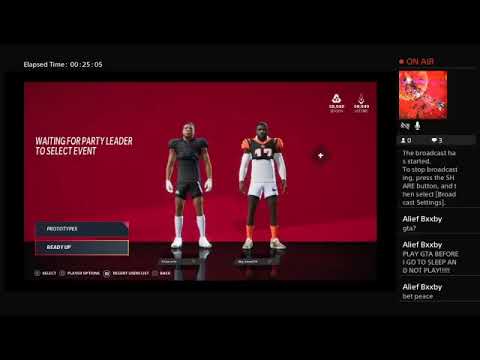The image is a screenshot from a video game, capturing a moment on the game interface. The elapsed time displayed is 00:25:05, and text on the screen reads: "Waiting for party leader to select event." Two athletic figures, resembling football players, are positioned centrally in the image. One player is dressed entirely in black, including a black jersey, black shorts, white socks, and white shoes. The other player wears a more colorful ensemble, featuring a black shirt with orange accents on the sides, a white undershirt with white sleeves, and white shorts.

Surrounding the characters are various buttons, presumably for game interactions, one of which likely allows players to indicate their readiness. To the side, a group chat section is visible, showing three messages. Above the chat, an "On Air" indicator is illuminated in red, accompanied by a microphone icon, indicating a live broadcast. The overall background of the interface is predominantly black, with the central area being more colorful, typical of a television screen focused on the game content.